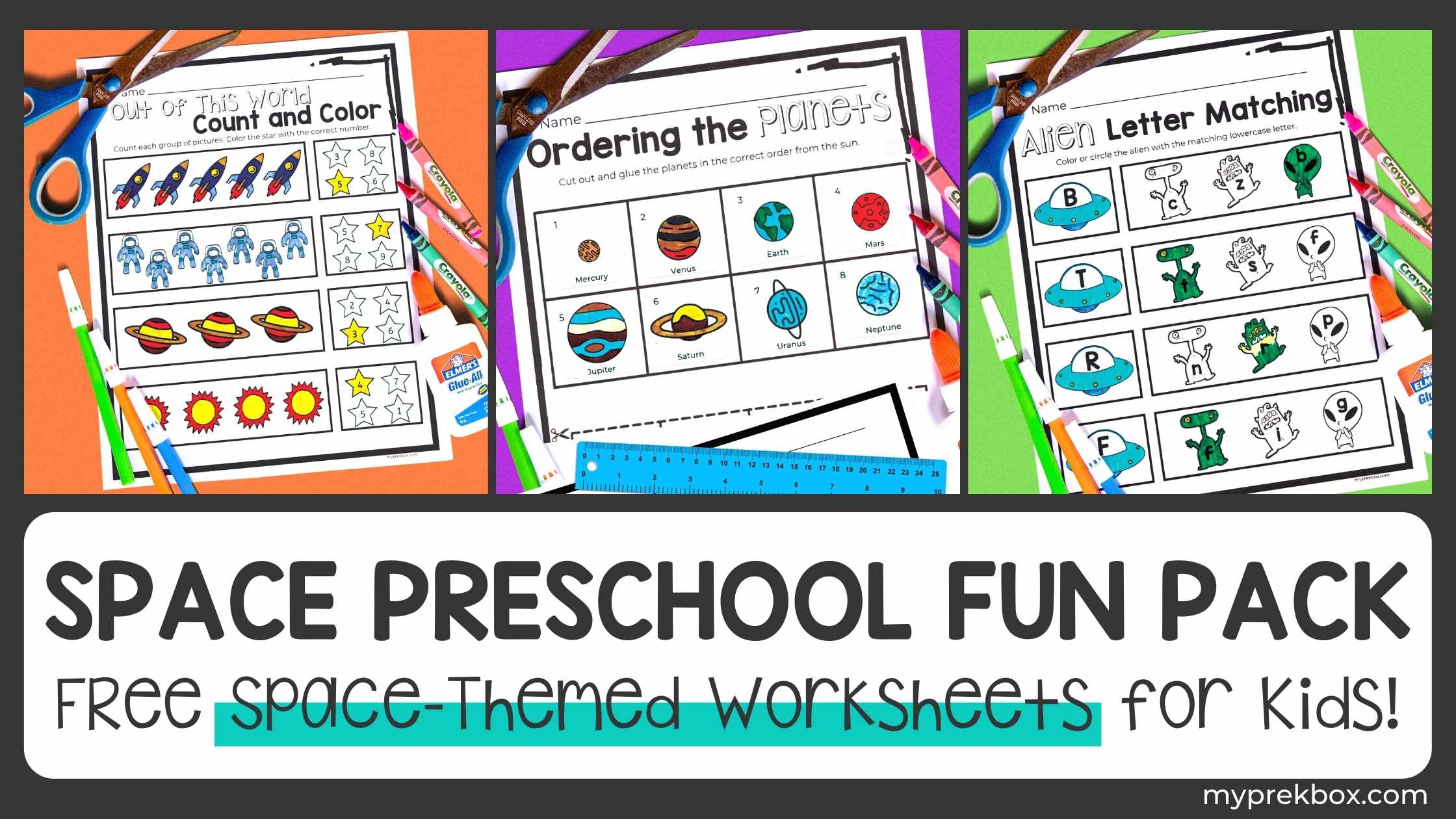The image is an advertisement for a "Space Preschool Fun Pack" from MyPKBox.com, featuring free space-themed worksheets for kids. It showcases three vividly colored worksheets positioned side by side. The first worksheet, set against an orange background, is titled "Out of This World Count and Color" and includes images of space objects like spaceships, astronauts, and suns, along with crayons and scissors. The middle worksheet, with a blue background, is labeled "Ordering the Planets" and displays various planets, a blue ruler, and additional crayons and scissors. The third worksheet, on a green background, is named "Alien Letter Matching" and features UFO and alien illustrations alongside crayons, markers, and scissors. A white banner beneath the worksheets announces "Space Preschool Fun Pack: Free Space Themed Worksheets for Kids" in black font, with "space themed worksheets" highlighted by a blue stripe. The bottom right corner of the image prominently displays "MyPKBox.com".